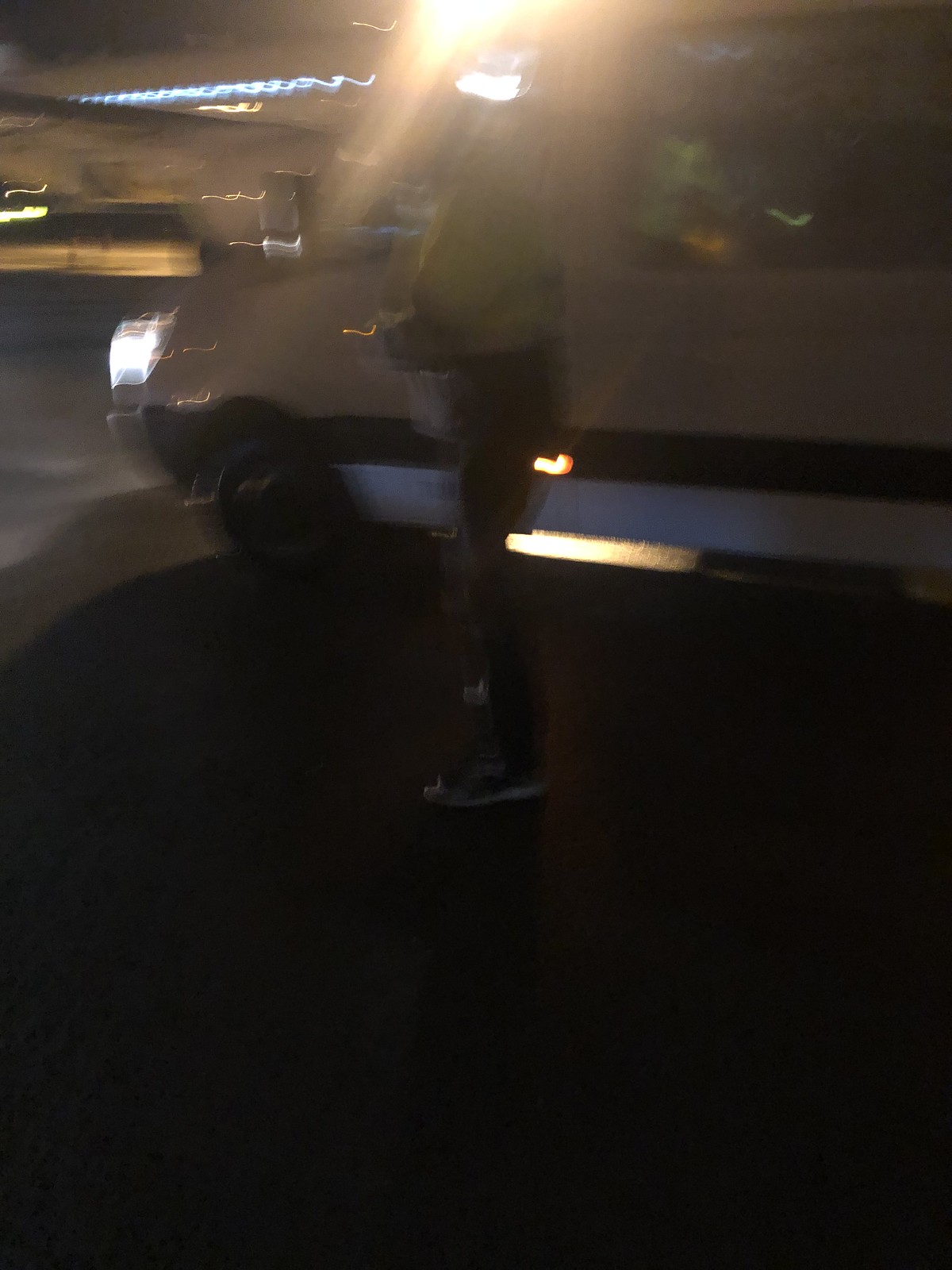In this dimly lit, blurry photograph, we find ourselves potentially inside a parking ramp. The image reveals a dark, shadowy ambiance with indistinct details. In the foreground, a person dressed in dark pants and a lighter-colored top stands partially illuminated yet mostly obscured. The bright headlights of a white vehicle with a black stripe penetrate through the gloom, casting light on the person but blurring their features. Above their head, a distorted smear of light dramatically overshadows them, creating intense rays that wash out much of their upper body. In the background, the top left corner hints at another vehicle, equally streaked and fuzzy, blending into the murky surroundings. Additional sources of dim, indistinct light streak across the top of the photo, while the bottom remains enveloped in darkness. The overall scene creates a mysterious and almost disorienting atmosphere, with light fighting against the encompassing shadow.